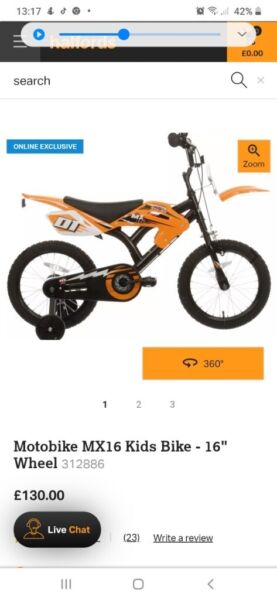In the image viewed on a mobile device, we see a product listing, likely from a website or app, showcasing a bike. 

In the upper left-hand corner of the screen, the time displayed is 13:17, accompanied by several icons, including a recognizable TikTok icon. There is a circular icon and another icon resembling an anchor. On the far right of the screen, indicators for an alarm clock, data signal, Wi-Fi signal, and battery status show a 42% battery life next to an almost depleted battery icon.

Beneath these indicators, there is an oval-shaped white band featuring a blue play button and a volume indicator set at the midpoint. Partially obscured by this band is a black banner reading "Halfords," with an orange section also partially hidden. Below this, there are search functionalities and an "Online Exclusive" tag.

The main image presents an orange and black, dirt bike-looking bike labeled "Motobike MX-16 Kids Bike" with a 16-inch wheel size. The product details include a reference number, 312-886, and a price of £130. Additional options on this listing include a "Live Chat" feature, and links to 23 reviews or an option to write a review.